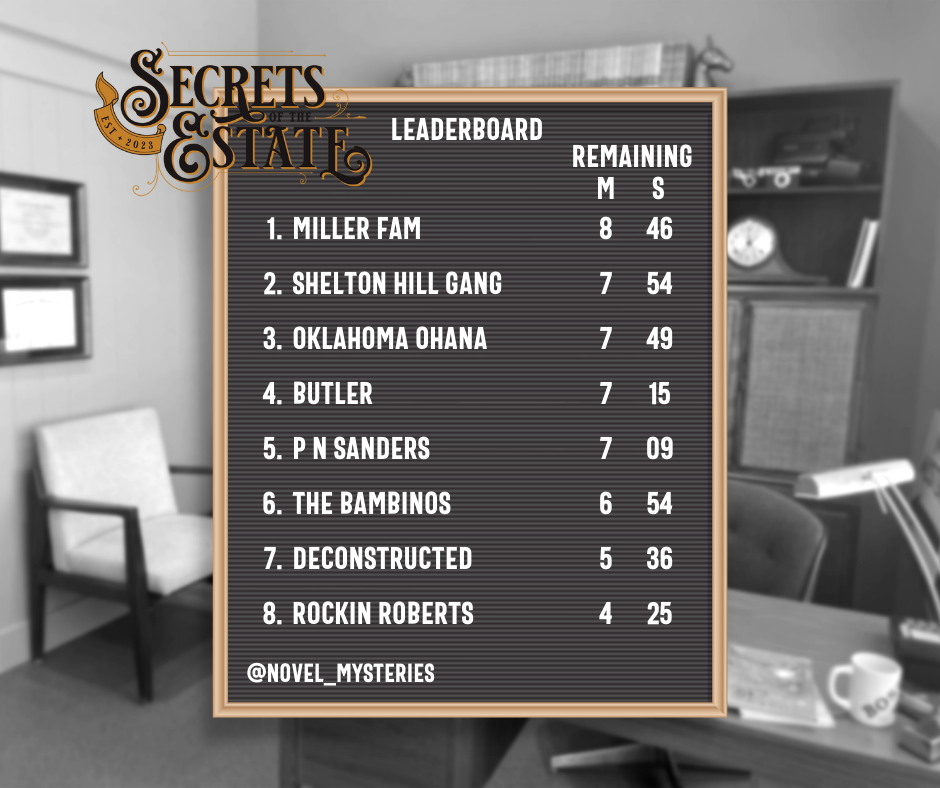This image depicts a black-and-white photograph of what appears to be an office, likely that of a professional such as a real estate agent, lawyer, or accountant. The office is somewhat out of focus in the background, with notable details such as a desk featuring a white coffee mug with the word "Boss" embossed on it and a desk lamp. To the right, there is a shelving unit with various items, including a mantle clock. Adjacent to the shelving are two framed certificates hanging on a plain gray wall, under which stands a side chair with wooden arms and legs. 

Superimposed at the center of the photograph is a leaderboard belonging to an organization called "Secrets of the State," established in 2023. This leaderboard lists eight different teams or groups with their standings and performance statistics. The top team is the Miller Family, followed by the Shelton Hill Gang, Oklahoma Ohana, and the Butler team, among others. The leaderboard is flanked by two columns with the headings "remaining M" and "S." Additionally, a social media handle "@Novel_Mysteries" is displayed at the bottom of the board. The only colors breaking the monochrome palette are tan and mustard hues outlining the leaderboard.